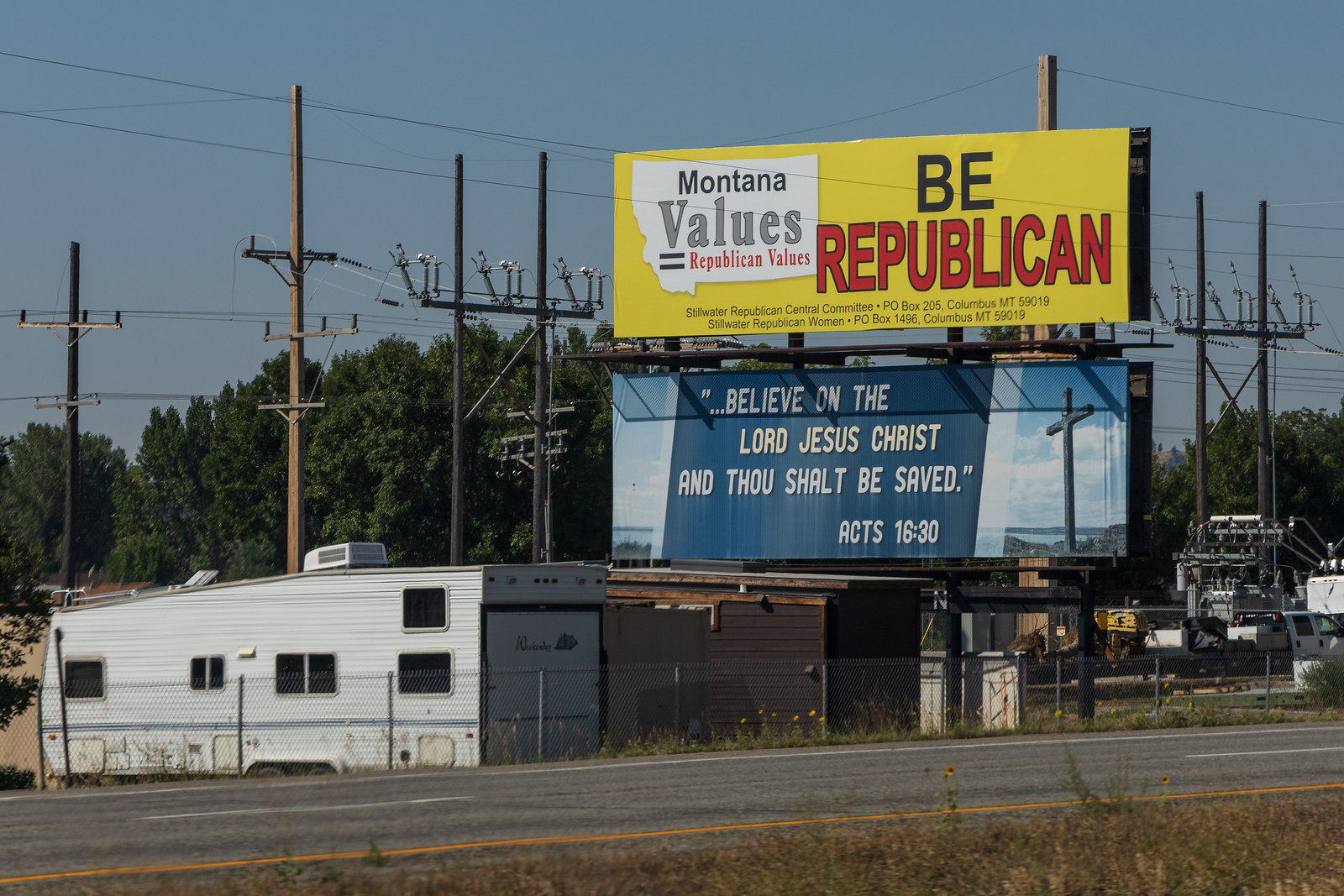Across a horizontal, two-lane gray road, a detailed scene unfolds. On the far side of the road, a tall chain link fence encloses a multifaceted area. Behind this fence, a white trailer or RV is parked at an angle, prominently featuring an air conditioner vent atop its roof and five visible windows on its left side. Adjacent to the trailer on the right, there is a dilapidated brown tar paper shack, indicating a state of disrepair.

Further to the right, a network of utility poles rises high into the sky, each adorned with transformers, signposting this area as a hub for electricity production or servicing. Central to the image are two billboard signs, one stacked above the other. The top billboard reads "Be Republican" in bold red and black letters, accompanied by a white banner on the left side. Below it, in a mix of light blue on the edges and dark blue in the center, the lower billboard proclaims in white text, "Believe in the Lord Jesus Christ, and thou shalt be saved. Acts 16:30."

To the far right of the scene, a building's structure peeks into view, likely the office for personnel working within the fenced compound. This complex tapestry of elements provides a glimpse into a location where public messages, utility operations, and varied structures coexist.